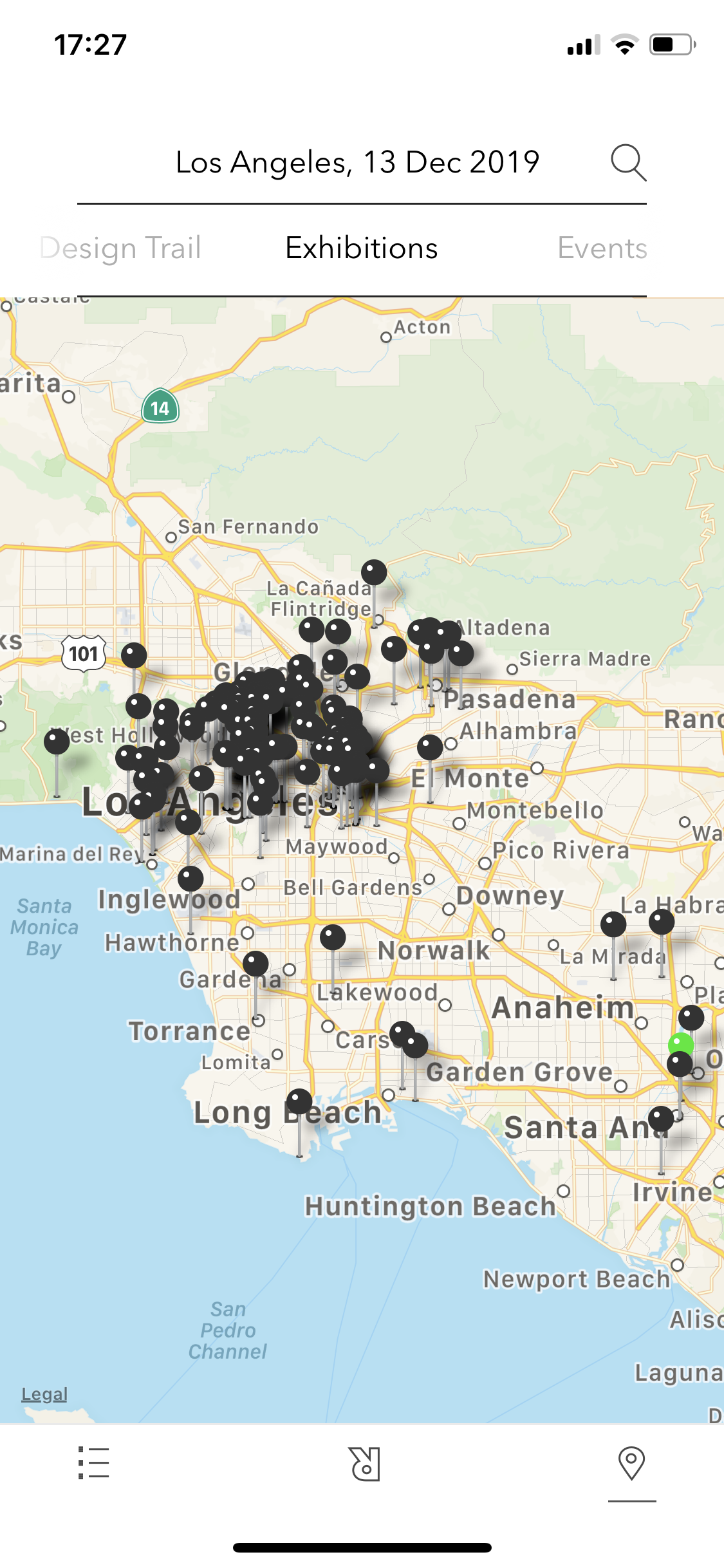The provided image is a screenshot of an iPhone display showing a Google Maps interface. At the top of the screen, the status bar indicates the time is 17:27 in 24-hour military format. To the right of the time, the battery icon shows it is halfway drained, there is a Wi-Fi symbol with two out of three bars, and the cellular signal strength displays three out of four bars.

The map interface appears to have a search result for "Los Angeles, 13 December 2019," suggesting the user is possibly looking for events or locations relevant to that date. The map is populated with black pins indicating various exhibitions, likely targeting a tourist or someone interested in cultural or local events.

At the bottom of the screen, there are typical map settings symbols, including an unexplained icon resembling an upside-down "R." This icon's function is unclear from the screenshot alone.